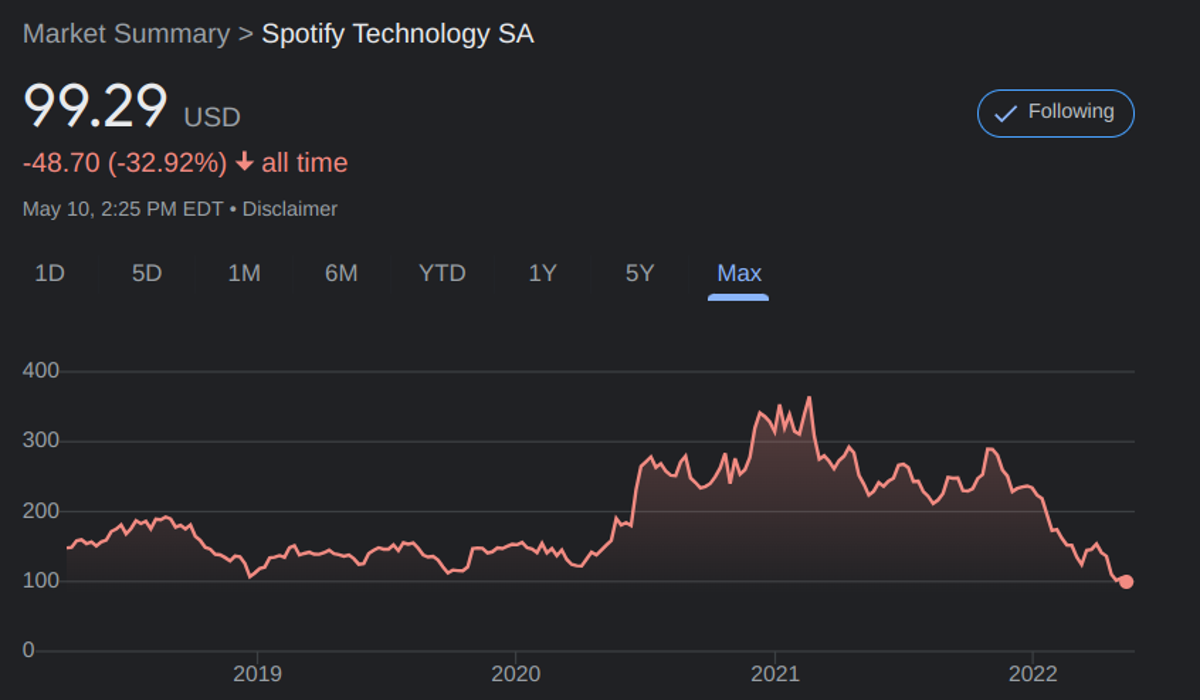This image is a market summary chart for Spotify Technology S.A. The background of the image is entirely black, providing a stark contrast to the text and graphics. At the top right corner, there is a blue "Following" button with a white checkmark inside it, indicating that the user is following this stock.

The title "Market summary" is displayed in gray text, while "Spotify Technology S.A." is prominently shown in white. Below the company name, the current stock price is listed as "99.29 USD," accompanied by a significant negative change, "-48.70 (-32.92%)," displayed in parentheses indicating a decrease, and noted as "down all time."

The chart below the text spans from the years 2019 to 2022. A red line represents the stock's performance over this period. Initially, the line hovers between $100 and $200. Around 2020, the stock price begins to rise sharply, peaking close to $400. After this peak, the price declines steadily, returning to just below $100 by the end of the period shown. The label "max" is situated beneath the chart, highlighted with a blue underline, possibly indicating the data range being displayed.